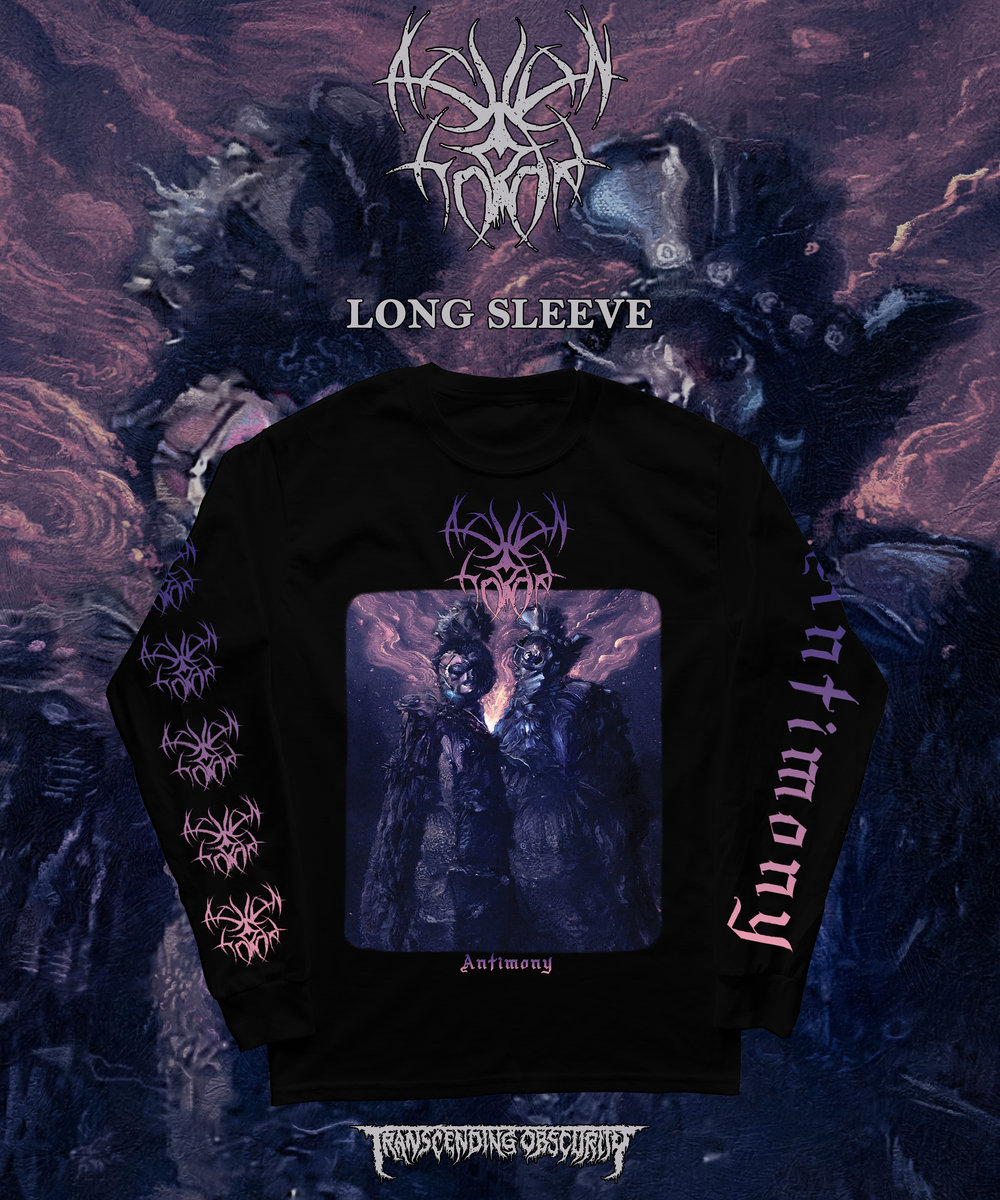The image portrays a dark, textured poster dominated by blue, black, purple, and gray hues, with intricate swirls and detailed imagery creating a complex background. At the top, a white logo resembling intertwined branches precedes the word "Long-Sleeve" in white. Centrally featured is a black long-sleeve t-shirt adorned with a surreal and eerie design. The design includes two humanoid figures with bird masks and costumes, rendered in dark, blotted tones consistent with the poster's color palette. The t-shirt also displays the word "Antimony" in a unique font, with the same lettering style extending to the sleeves. In stark, horror-inspired white letters near the bottom of the poster, it says "Transcending Obscurity," enhancing the ominous feel of the entire composition.